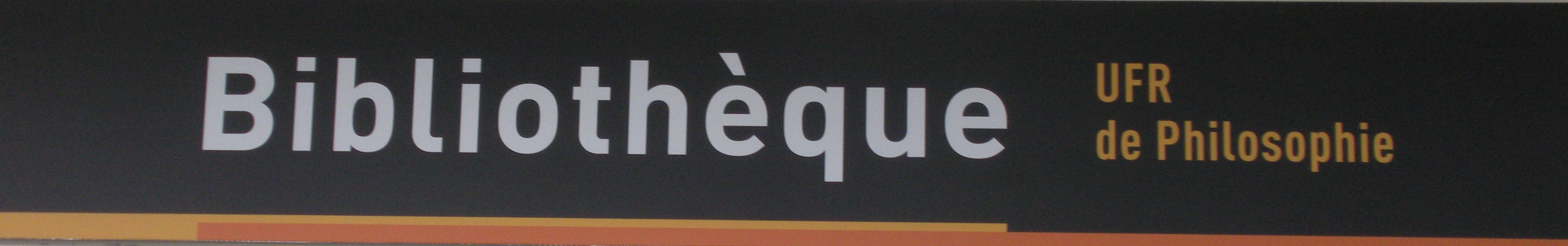The image features a zoomed-in view of a rectangular black sign, reminiscent of a billboard. Beneath the black rectangle are two horizontal lines: one beige and one orange. In the same beige color, towards the right side of the sign, the text reads "UFR Day Philosophy," suggesting it might be in Spanish. On the left center, the word "Bibliothèque" is prominently displayed in white letters, with an acute accent over the first 'e,' spelled out as B-I-B-L-I-O-T-H-È-Q-U-E.